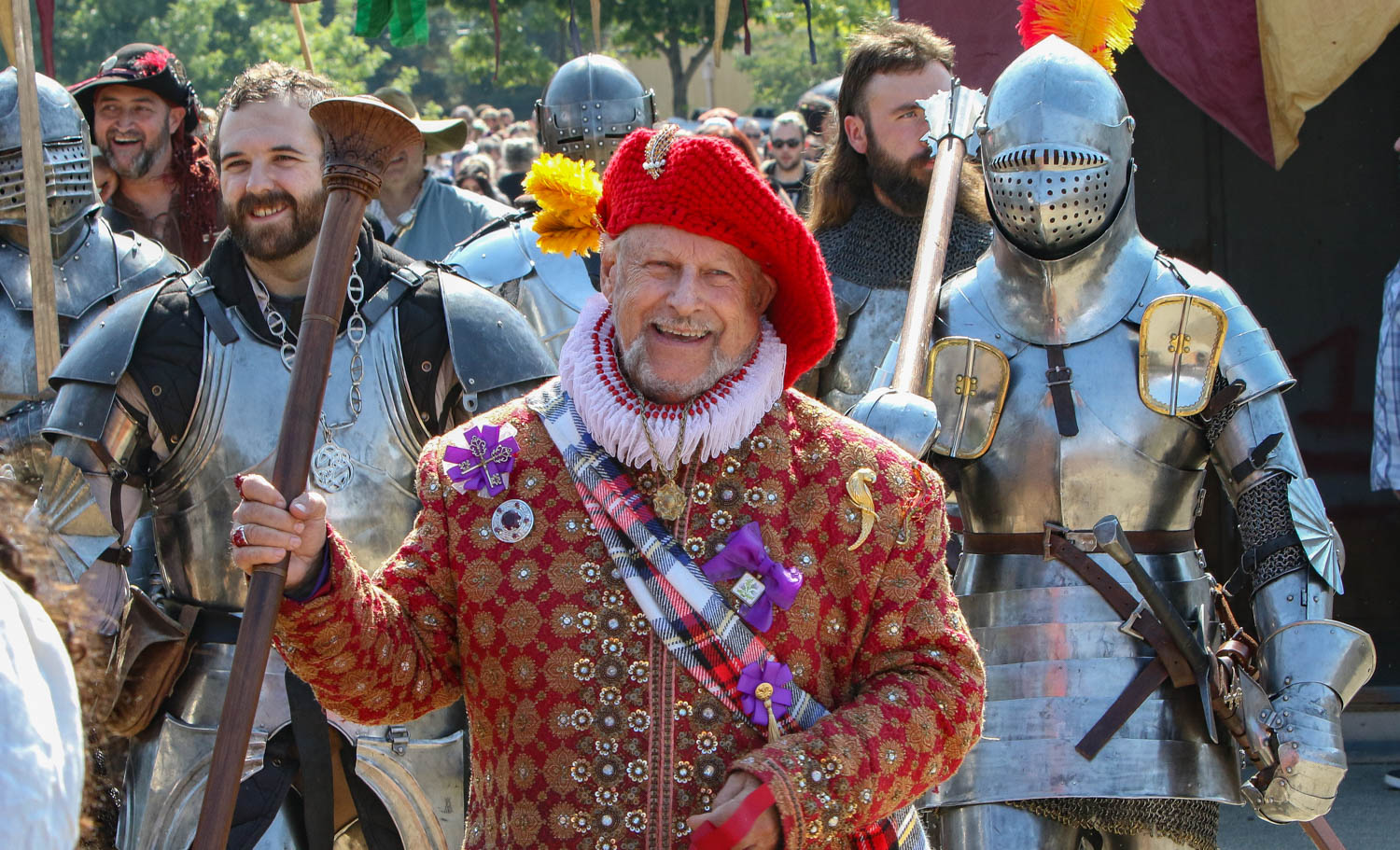The image captures a lively scene reminiscent of a Renaissance festival. At the center of the horizontally aligned rectangular picture stands an older man, distinguished by his white mustache and beard. He is adorned in an elaborate red and gold patterned coat with ornate details and a fringe resembling a turtleneck around the neck. Complementing his outfit, he wears a red knitted cap decorated with gold accents and yellow feathers trailing from the back, resembling a long beret.

Surrounding him is a vivid crowd, primarily composed of men dressed as Renaissance soldiers or knights. Many of these men are clad in silver armor with accents of black around the shoulders, and a few feature gold highlights. Some of the knights wear helmets that cover most of their faces except for the eye and mouth openings, and they hold weapons like swords and staffs. The man behind him to the right has his helmet on, while another on the left has removed his helmet, revealing a metal-clad ensemble. The scene suggests a festive procession, possibly a parade, with onlookers gathered to watch the spectacle unfold.